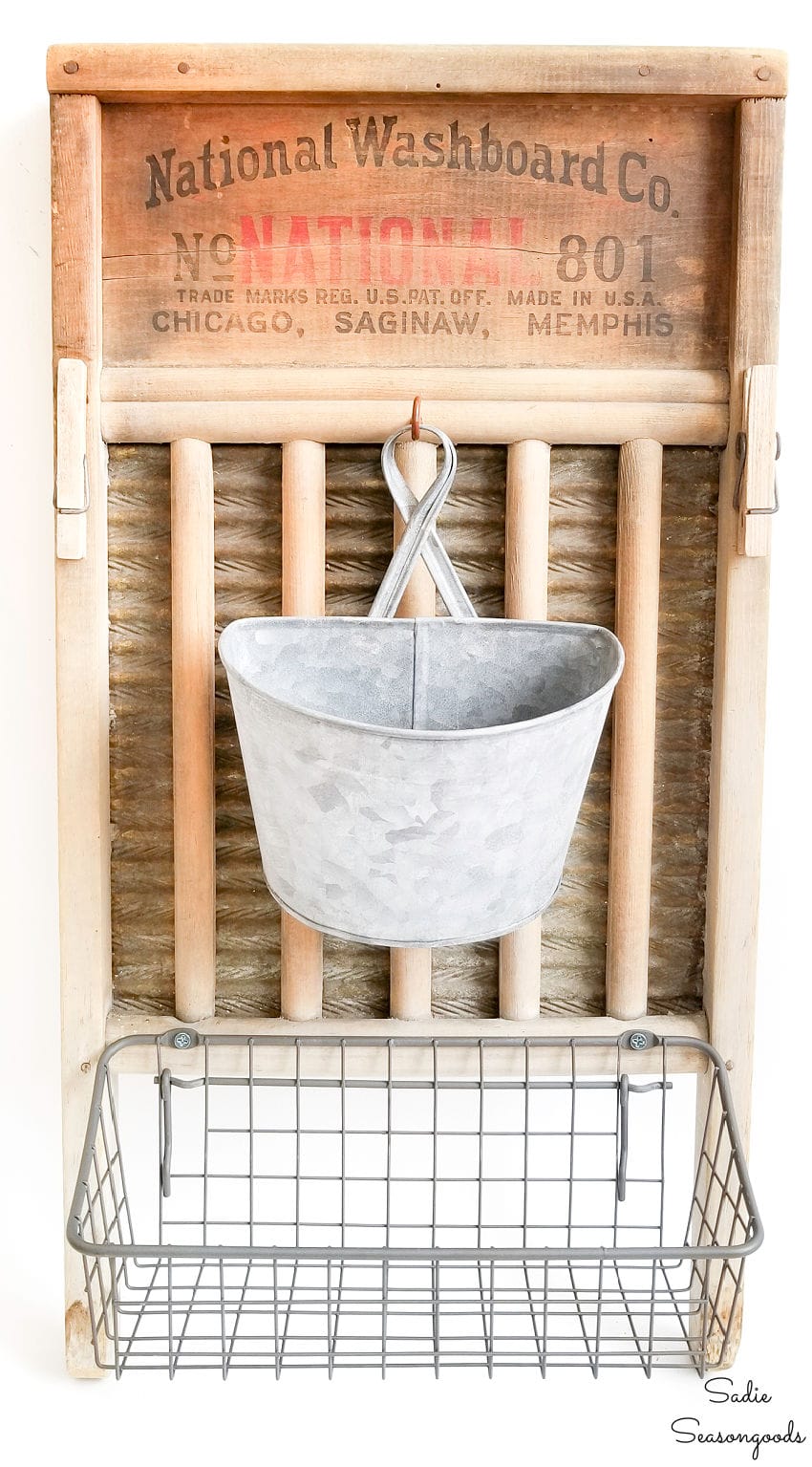This vertically oriented photograph features a realistic and nostalgic depiction of an old-fashioned washboard, a once-essential tool for laundry. The washboard is prominently marked with "National Washboard Company, National 801" in black and red fonts, along with other details such as "Trade Mark Reg, U.S. Pat Off," and locations "Chicago, Saginaw, Memphis." The wooden board is paired with a piece of corrugated metal typically used for scrubbing clothes. Suspended from the washboard is a well-worn, oval metal bucket with a handle, measuring approximately 12 inches by 12 inches, adding to the antique ambiance. Below this setup, a metal wireframe basket, roughly two feet wide and one foot deep, completes the setting. The entire arrangement is set against a white background, highlighted by a small, elegant signature in black font at the bottom right, which reads "Sadie Season Goods." This signature suggests that the photograph is a carefully curated artistic piece, celebrating the charm of vintage utility objects.